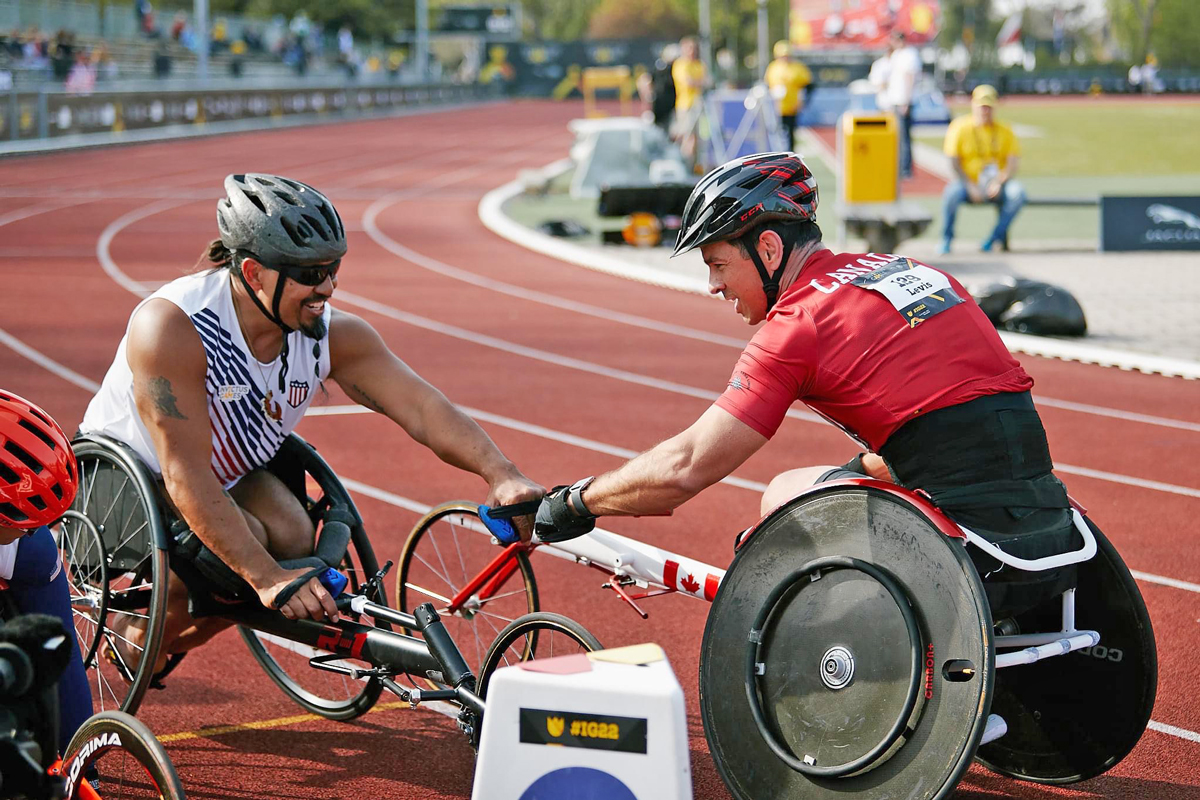This detailed photograph captures the spirited moment of two male athletes in a wheelchair racing event, taken on an outdoor red running track. The image shows the two jubilant athletes fist-bumping near the race's finish line, celebrating their accomplishments. 

The athlete on the right is dressed in a striking red outfit with the number 129 displayed on his chest and a black back brace. His gear includes a bike helmet, and his three-wheeled white wheelchair prominently features a Canadian flag on the frame. This man is smiling, exuding a sense of triumph and shared camaraderie with his fellow competitor.

The athlete on the left wears a sleeveless white jersey with diagonal blue stripes and a matching bike helmet with dark glasses, also sporting a goatee beard. His three-wheeled wheelchair is black, and although there is something red attached to it, its exact detail remains unclear. Both men exhibit muscular arms, emphasizing their athletic prowess.

In the backdrop, the image captures the curve of the red track, sparsely populated stands, and a few racing officials in yellow. An additional athlete is barely visible in the lower-left corner, observing the fist bumping scene. The background elements, including the spectators and referees, are slightly blurred, drawing clear focus to the two main athletes and their moment of celebration.